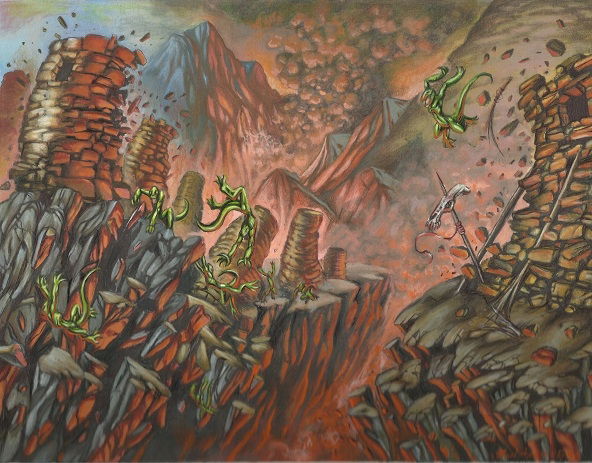In this chaotic and vividly detailed painting, a hellish, volcanic landscape unfolds with intense colors and dynamic movement. The backdrop is dominated by towering mountains and volcanoes spewing dark smoke into an orange and brown sky, lending an apocalyptic atmosphere to the scene. Rock formations and crumbling towers, constructed from irregular stones and bricks, are disintegrating under the apparent force of the eruptions. In the foreground, amidst the rubble and chasm filled with a reddened hue, surreal green creatures emerge. These creatures, resembling a hybrid of lizards and humans, leap and claw through the air with oblong heads, sharp teeth, long tails, and talon-like feet. Their fluorescent greenish-yellow bodies contrast starkly with the dark volcanic landscape. Some creatures appear to be attacking, their poses frozen in mid-leap or tumbling down rocky embankments, while others climb or fall from the collapsing cliffs. The overall scene is immersive and ominous, capturing the chaos and danger of this fantastical world.